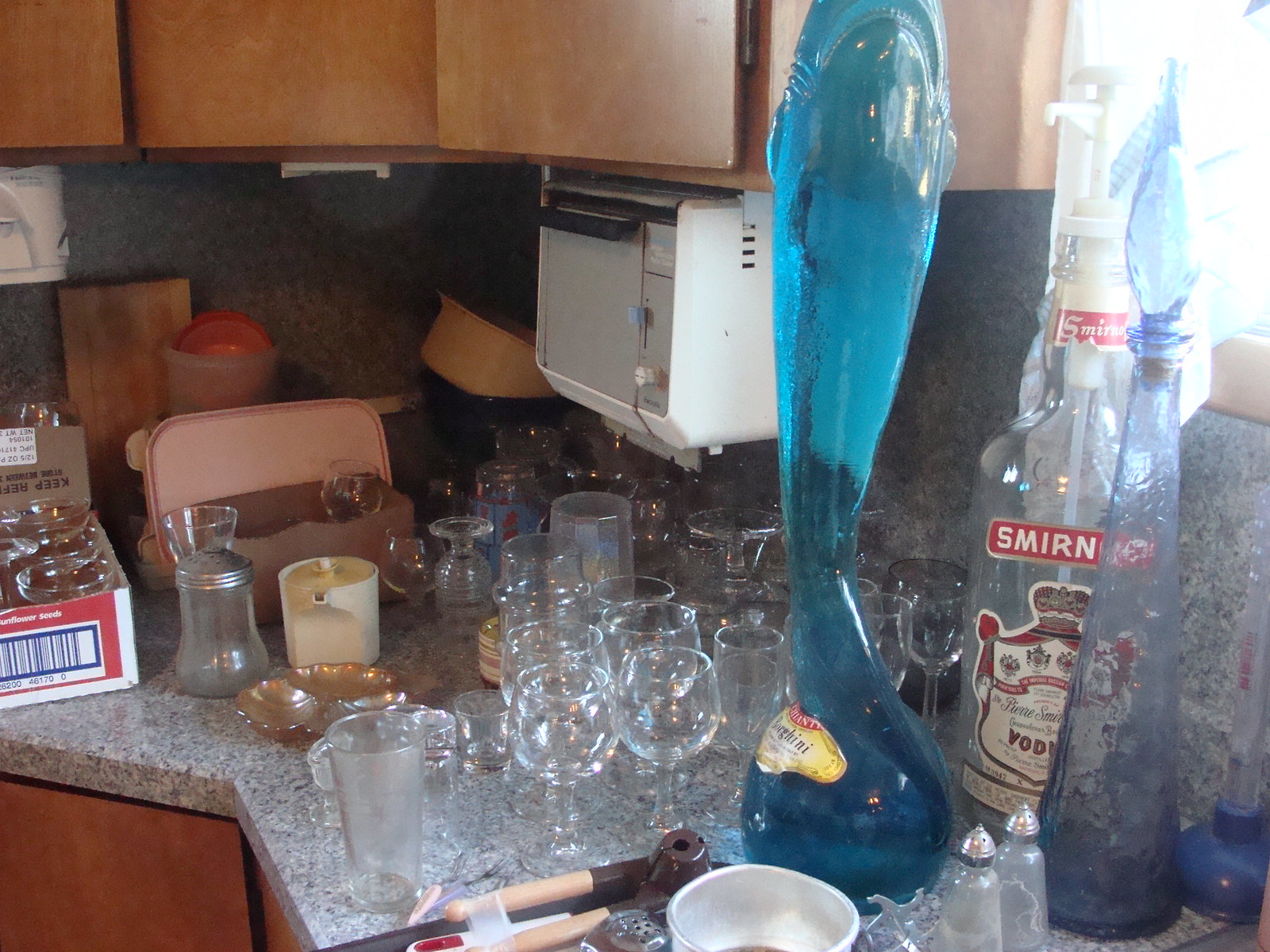This detailed photograph captures a close-up view of a corner section of a modern kitchen counter, featuring a diverse array of glassware and other intriguing items. The kitchen cabinets, though not the primary focus, are a medium brown wood with a handle-less design, contributing to the kitchen's contemporary aesthetic. 

The white granite counter is dotted with busy gray flecks, lending it a textured appearance. At the center of this scene lies an assortment of clear drinking glasses, each with its unique shape and purpose. Among them are deep-bellied wine glasses, slightly frosted beer glasses, standard water glasses with built-in grips, a champagne flute-shaped wine glass, and another frosted glass with an octagonal exterior surface.

Adding to the collection are some wide champagne glasses stored in a cardboard box, suggesting preparations for packing or storage. Nestled nearby is a salt or pepper shaker along with a champagne-colored candy treat tray. A tall blue decorative glass container with a delicate, fluted stopper adds a splash of color and elegance to the setting.

Prominent within this array is a bong alongside a lighter on a tray, hinting at recreational use. A large empty bottle of Smirnoff vodka, fitted with a pump, raises curiosity about its specific use. This eclectic mix of glass items and kitchen accessories paints a vivid picture of a busy, yet intriguing kitchen space.